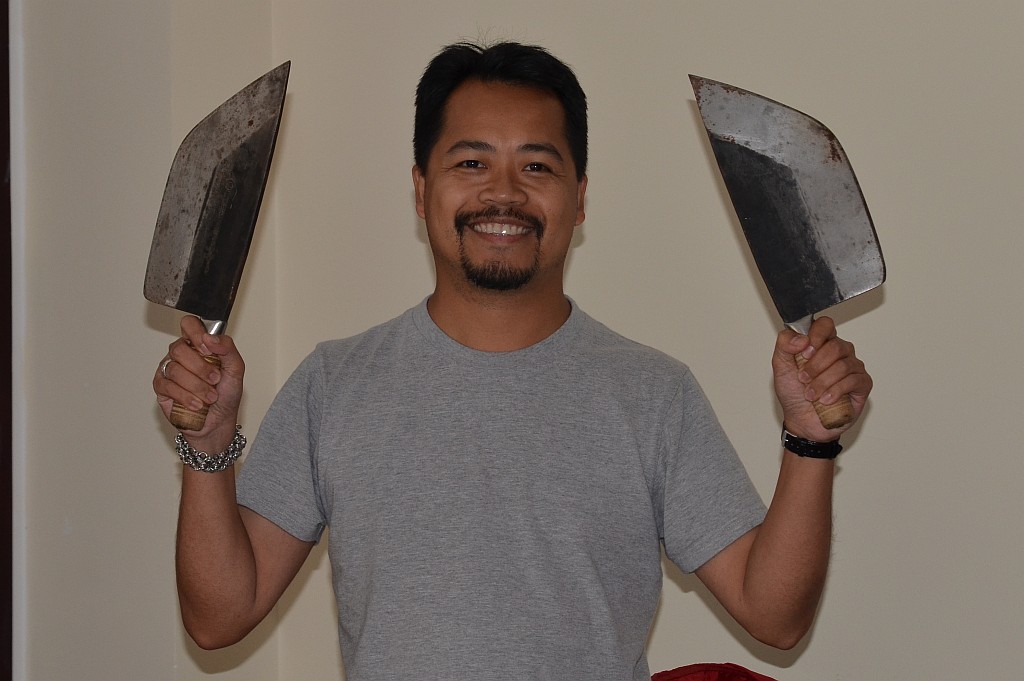This photograph features an Asian man, likely in his 30s or 40s, posing joyfully for the camera. He's sporting short, black hair and a black goatee, along with a gray t-shirt devoid of any logos or graphics. With a cheerful smile that reveals his teeth, he's holding up two large, weathered cleavers that appear to have wooden handles and show signs of rust, suggesting they are not used for cooking. One cleaver is held in each hand near his head. His right wrist is adorned with a silver metal bracelet, while his left wrist sports a black wristwatch. The background is plain, with a yellowish tint, adding no distraction to the focus on the man and his cleavers. The image captures him from the waist up, showcasing his animated and engaging pose.